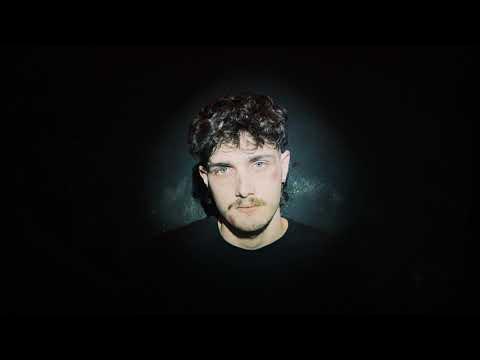A man with fair skin and short, curly, dark hair, styled in a possible mullet with curls around the nape of his neck, sits against a predominantly black background. His head is framed by a soft, white circular light, creating a halo effect that illuminates his face and part of his chest. He has symmetrical ears, dark eyebrows, and light-colored eyes—either grayish-blue or brown. His mustache is thin and sparse, appearing brownish-black, with a hint of chin hair visible. He is wearing a black shirt that blends into the shadowy backdrop, making it seem as though his head is emerging from darkness. The background, while primarily black, features subtle dark teal and white markings, reminiscent of distant stars or a cosmic scene. His head is tilted slightly to the left, and his gaze is directed straight at the camera.